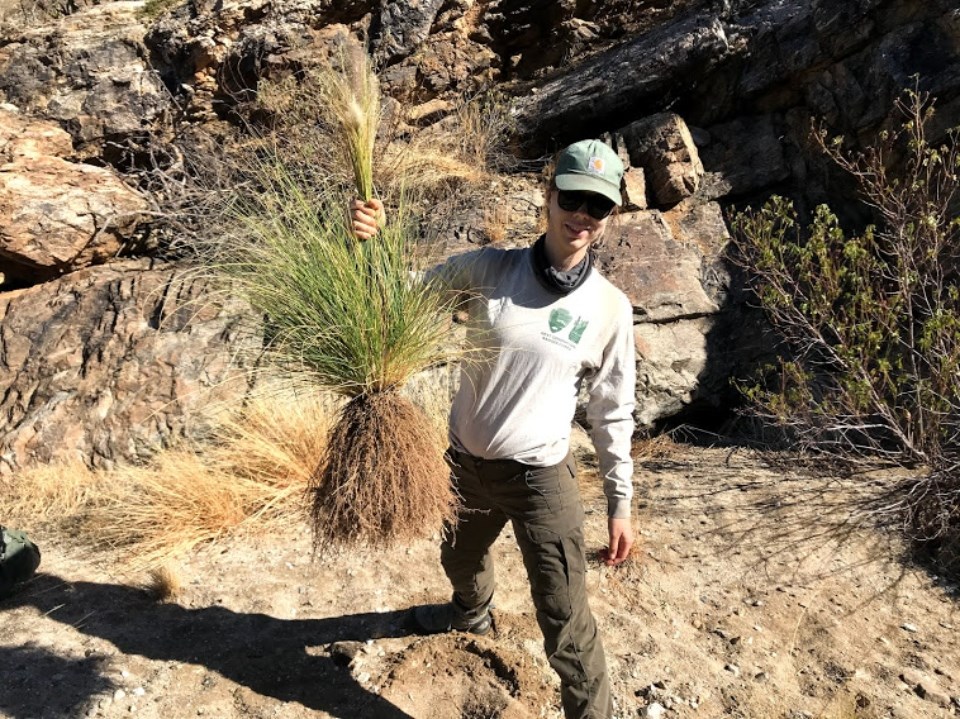In the foreground stands a man, poised in an uneven stance with his right foot forward and his left foot back. He dons a light green cap with a logo, black sunglasses, and a long-sleeved gray shirt featuring a green emblem. His brown cargo pants are paired with sturdy industrial boots suitable for rugged terrain. The man’s left hand is elevated, clutching a large bundle of grass with green blades and yellow seeds atop dark brown roots. His right hand hangs by his hip. He stands over a freshly-dug hole in light brown soil, the remnants of his harvest. Shadows stretch to his left, mirroring his actions against a backdrop of light gray and yellow rocks. The rocky cliff suggests a desert ecosystem, with scattered trees growing among the layers of stone. A solitary strawberry peeks into the frame from the right, adding a touch of color to the arid scene.